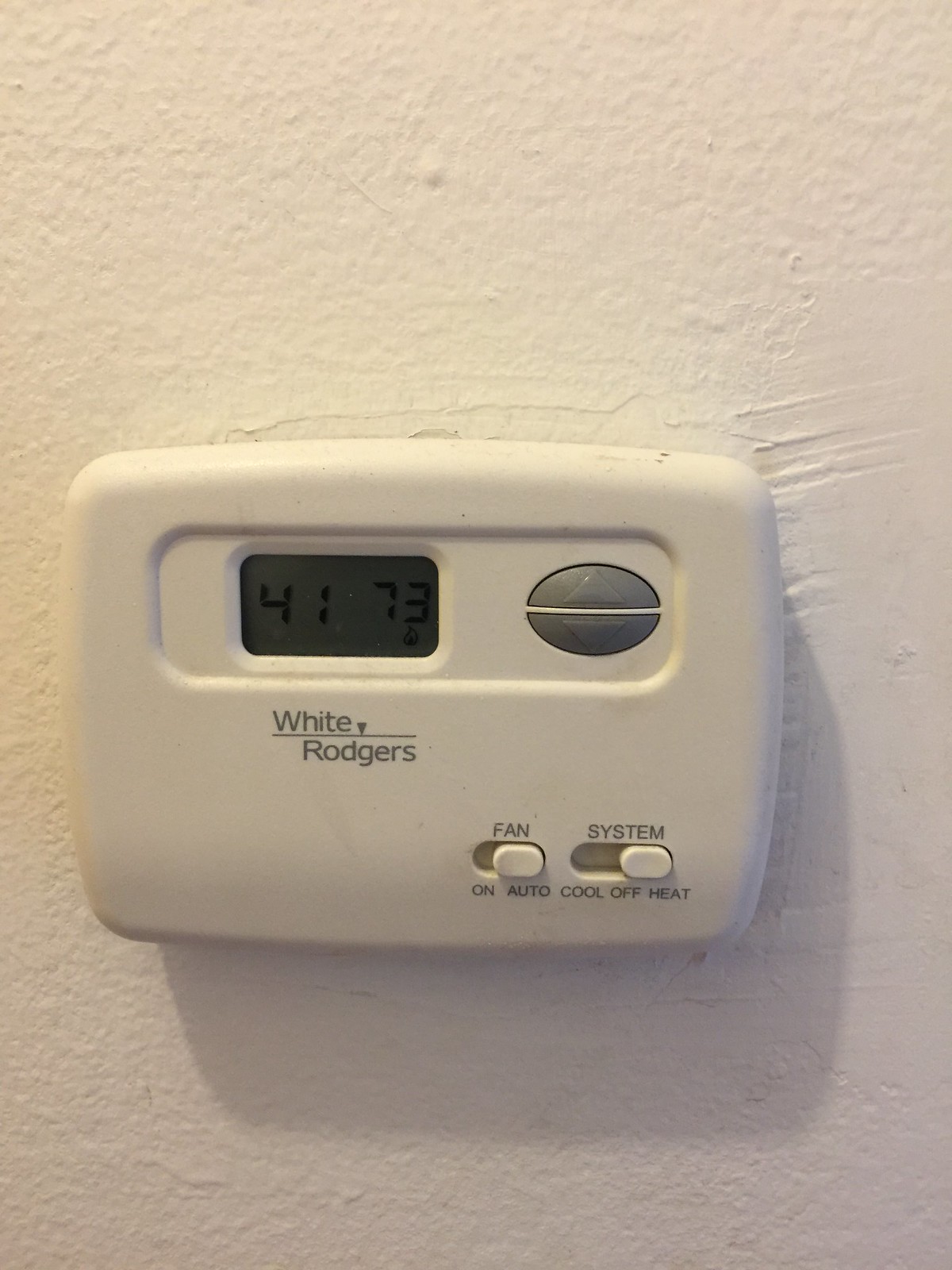A white plastic White-Rogers thermostat is mounted on a slightly textured, white-painted plaster wall. The paint exhibits noticeable brushstroke irregularities and small cracks around the thermostat installation area. The device appears old and somewhat dirty, with a notable accumulation of dust across the top surface. The digital display reads 73 degrees on the right side and 41 on the left, separated by a space. The fan is set to 'Auto,' and the system mode is configured to 'Heat.' A bright light illuminates the thermostat, casting a distinct shadow beneath and behind it. Adjacent to the display on the right, an up arrow and a down arrow button are visible, indicating basic temperature control functions.